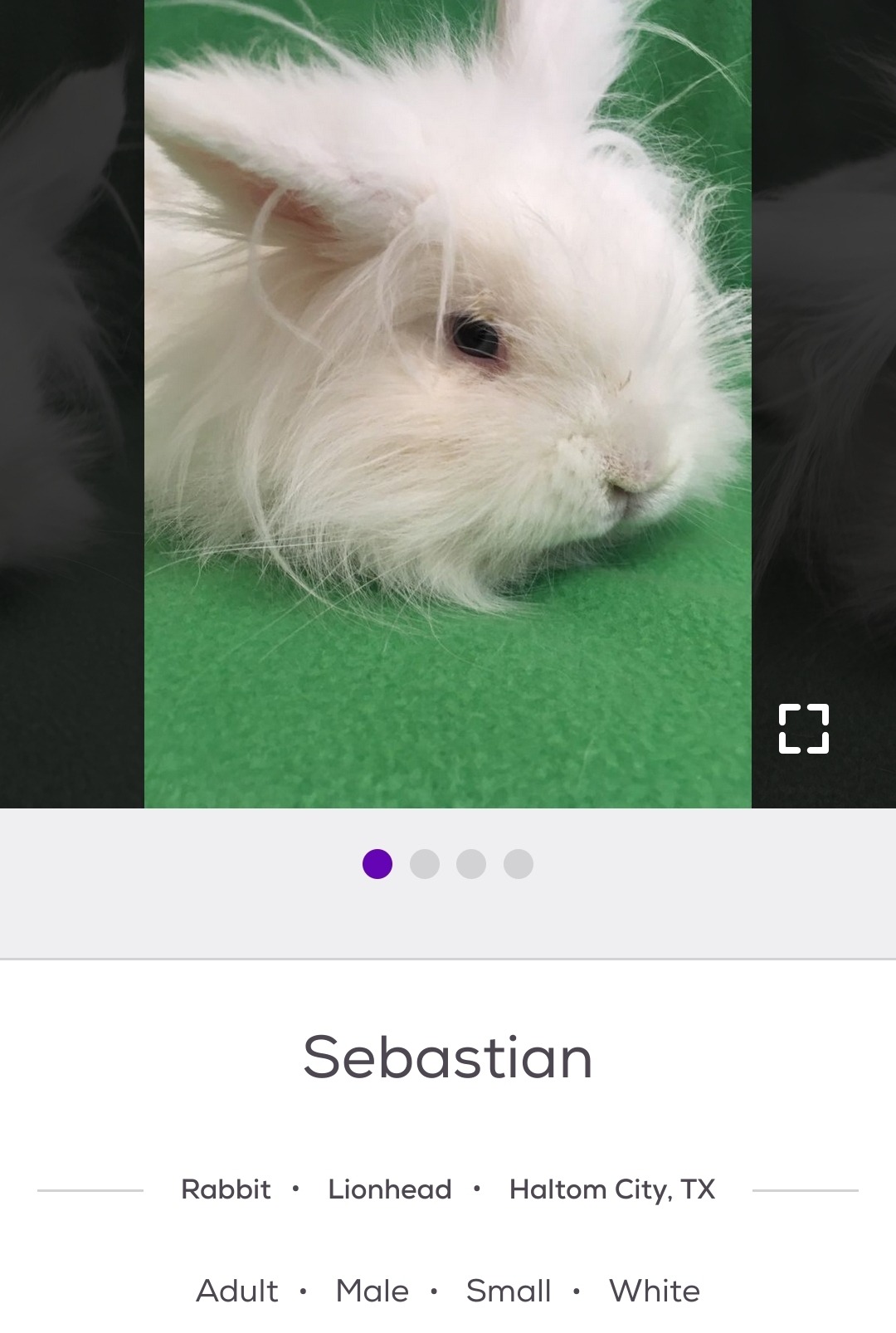The image is a screenshot taken from an unspecified website, as it lacks visible headers or footers identifying the site or company. Central to the image is a close-up, side-view photograph of a white rabbit named Sebastian. The focus is on Sebastian's head, highlighting his dark eye and soft fur, which is a grayish-white hue. Sebastian appears to have his chin resting on a green cloth-like surface. The image is bordered with a light gray strip at the bottom and black strips on either side. Below the photograph, set against a white background, is text providing details about the rabbit. The text reads: "Sebastian," "Rabbit," "Lionhead," followed by "Haltom City, Texas." Further descriptions indicate that Sebastian is an adult, male, small-sized white rabbit. This is the entirety of the information displayed about Sebastian in the image.